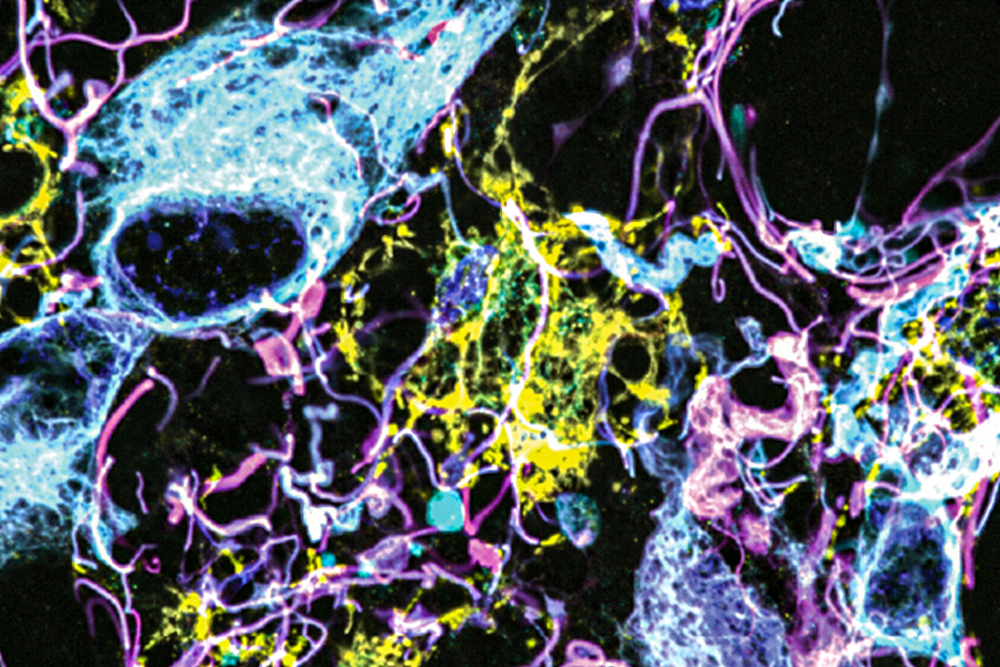The image is a vivid and highly abstract composition set against a black or dark purple background. It features a complex interplay of swirling lines and splotches, predominantly in bright blue, purple, and yellow hues. The blue areas are the most prominent, covering large portions of the top and bottom right sections of the image and extending through the painting in thin, swooping lines. Yellow is concentrated towards the center and the left, with smaller patches scattered around, while purple appears in wispy, smoke-like lines that weave through the composition. These colors mix together in a high-contrast, almost paint-splatter fashion, creating a dynamic and busy scene. The colors also incorporate touches of white, enhancing their intensity and giving the appearance that the entire piece could glow under the right lighting conditions.